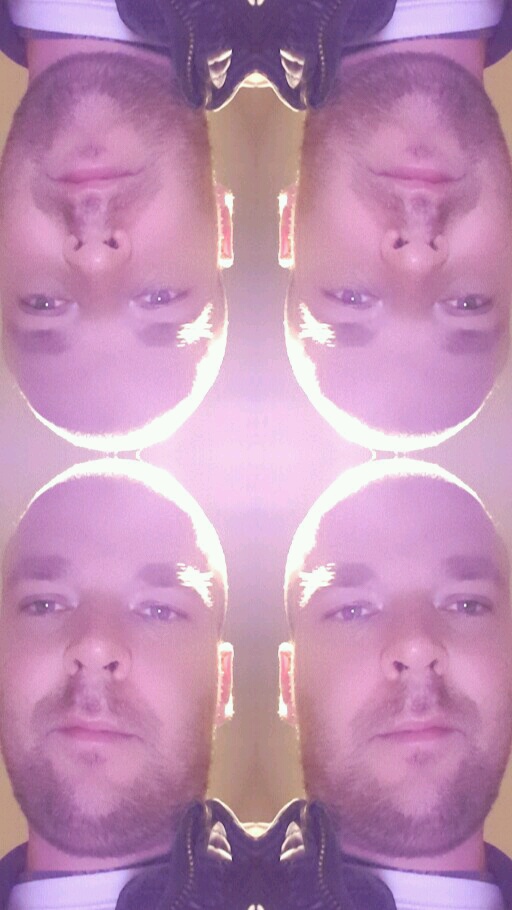The image is a meticulously edited photograph featuring a man who is repeated and mirrored, both horizontally and vertically, to create four distinct yet identical depictions of him. He appears to be in his early 30s, with a bald head, thick bushy eyebrows, blue eyes, a stubbly beard, and a mustache. He is dressed in a black denim jacket with an unfastened zipper, revealing a white t-shirt underneath. Towards the right of the jacket's zipper, there is a small cone-shaped detail. The man sports a neutral expression, looking directly at the camera in all iterations. The lighting, originating centrally behind the figure, highlights the top of his head in each mirrored image. This lighting accentuates the reflection effect, enhancing the symmetrical arrangement of the four mirrored images, with two faces oriented normally at the bottom and two inverted at the top, creating a visually balanced composition.